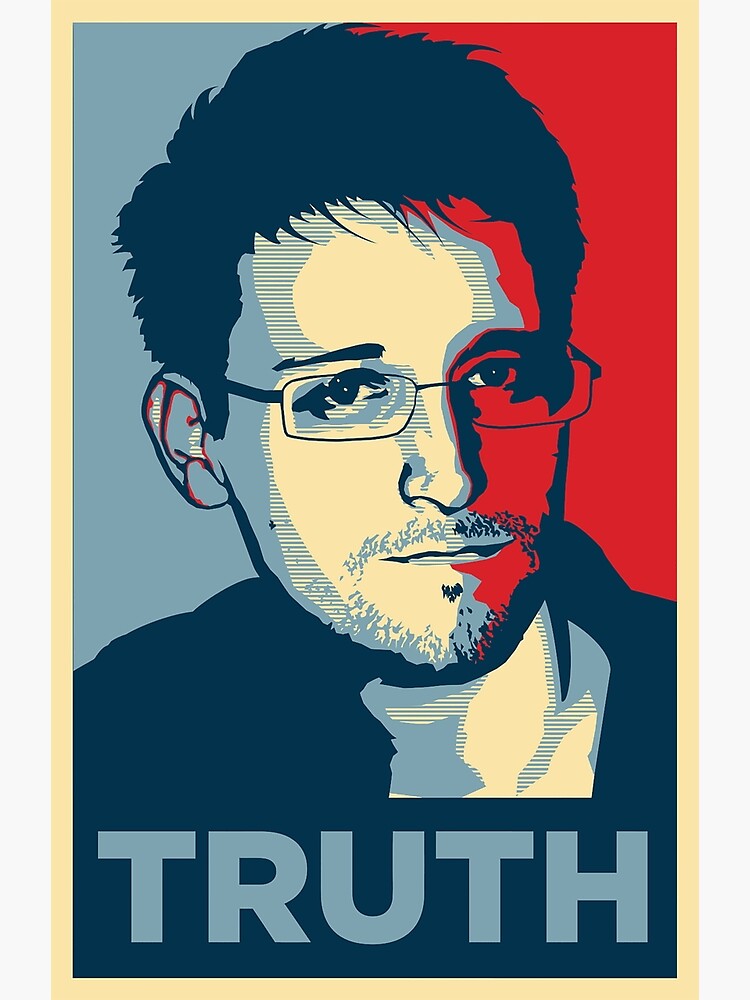This detailed drawing is a poster in a tall rectangular format, framed by a thin yellowish border. The background of the poster is split, with the left-hand side in a gray-blue hue and the right-hand side in a reddish tone, meeting in the middle to create a striking contrast. Dominating the poster is a stylized image of Edward Snowden, resembling the stencil style used in the famous Obama "Hope" poster. Snowden's face is divided, with the left side rendered in a blue-gray shade and the right side in red, emphasizing the duality of his controversial figure. He gazes directly at the viewer through glasses with rounded rectangular frames, and his facial features include messy, dark blue hair, a scraggly mustache, and a short goatee. He wears a dark blue shirt, further adding to the somber palette of the image. At the bottom of the poster, in large block, gray letters, the word "TRUTH" is prominently displayed. This artwork, likely intended as a political piece, visually encapsulates Snowden's role in revealing critical information from the NSA, blending elements of patriotism and dissent.